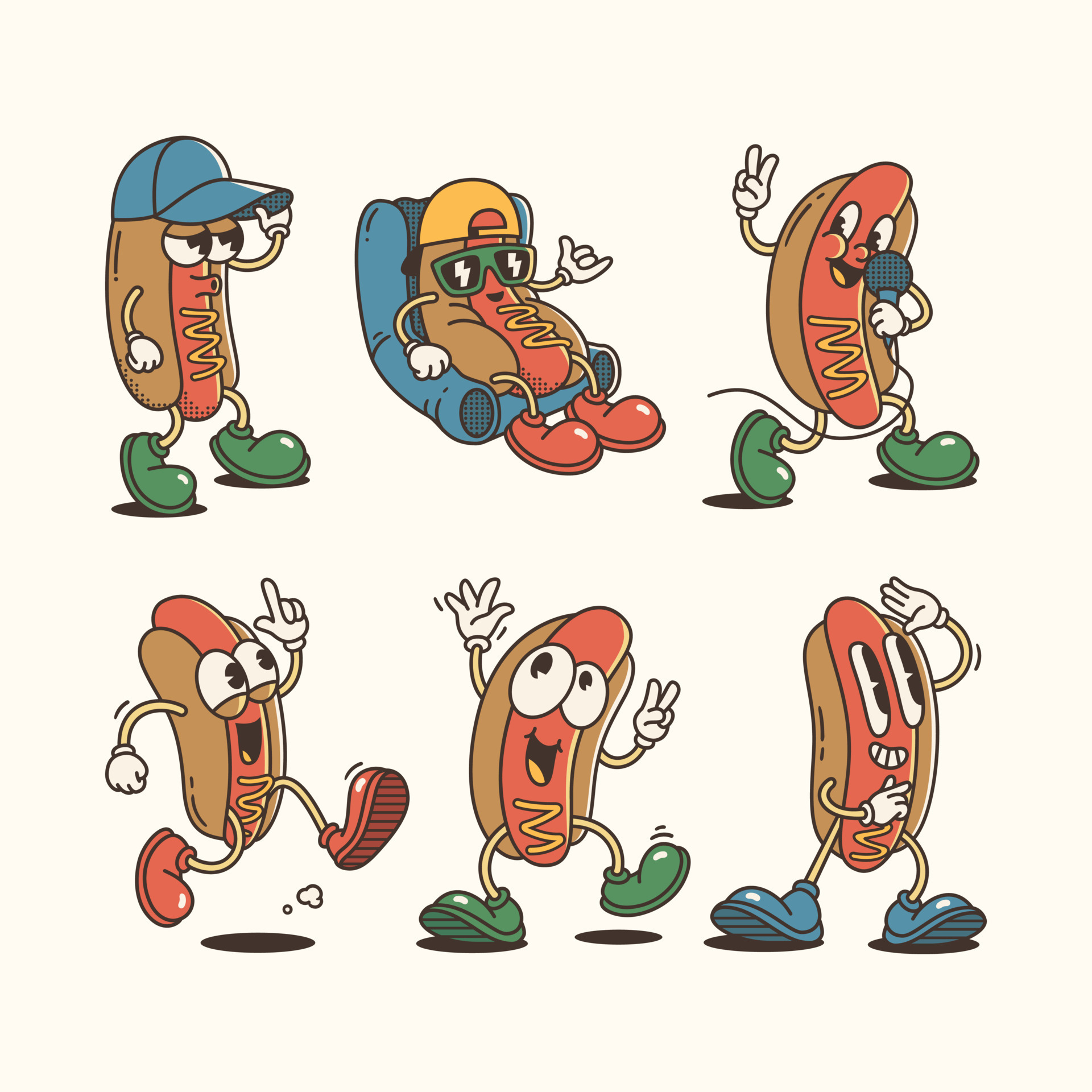This illustration showcases a lively ensemble of six animated hot dog characters set against a white background, arranged in two rows of three. On the top row, the character on the far left sports a blue cap and green shoes, with white mitten-like hands and googly eyes, its orange hot dog body adorned with a line of yellow mustard. To its right, a hot dog lounges on a blue chair, making a surfer gesture with a hand clad in a yellow backwards hat and green glasses. Completing the top row, the third character holds a blue microphone, flashing a peace sign with its fingers.

The bottom row starts with a dynamic character on the left that appears to be running and pointing with one hand, its mouth curled into a smile. Next, there’s a friendly hot dog waving one hand while making a peace sign with the other, wearing green shoes. The final character on the bottom right has a pair of elongated, oval-shaped eyes, one hand thoughtfully placed on its chin, and the other seemingly searching for something, all while grinning playfully. Each hot dog character adds a unique touch to this fun, spirited illustration with their colorful footwear — blue, red, or green shoes — and a dash of mustard on their bodies.